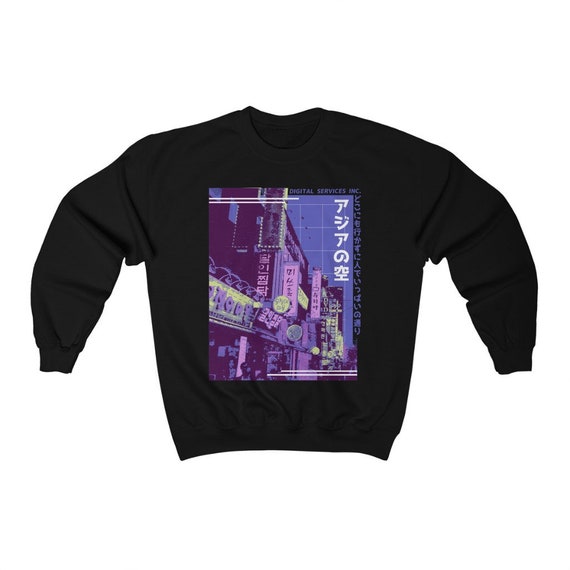The image showcases a black, long-sleeved, round-neck sweatshirt laid out on a completely white background, with its arms extended outwards. The focal point of the garment is a large, vertically rectangular graphic printed on the front. This graphic, taller than it is wide, depicts a city street scene with pastel hues of purple, yellow, indigo, lime green, and light gray, contributing to a vibrant yet faded aesthetic. The image features storefronts and billboards, suggesting an urban, possibly Asian cityscape, with various signs. Notably, there is text in the upper right corner of the graphic that reads "Digital Services Inc.," and a column of Japanese characters descends from the top right of the image.